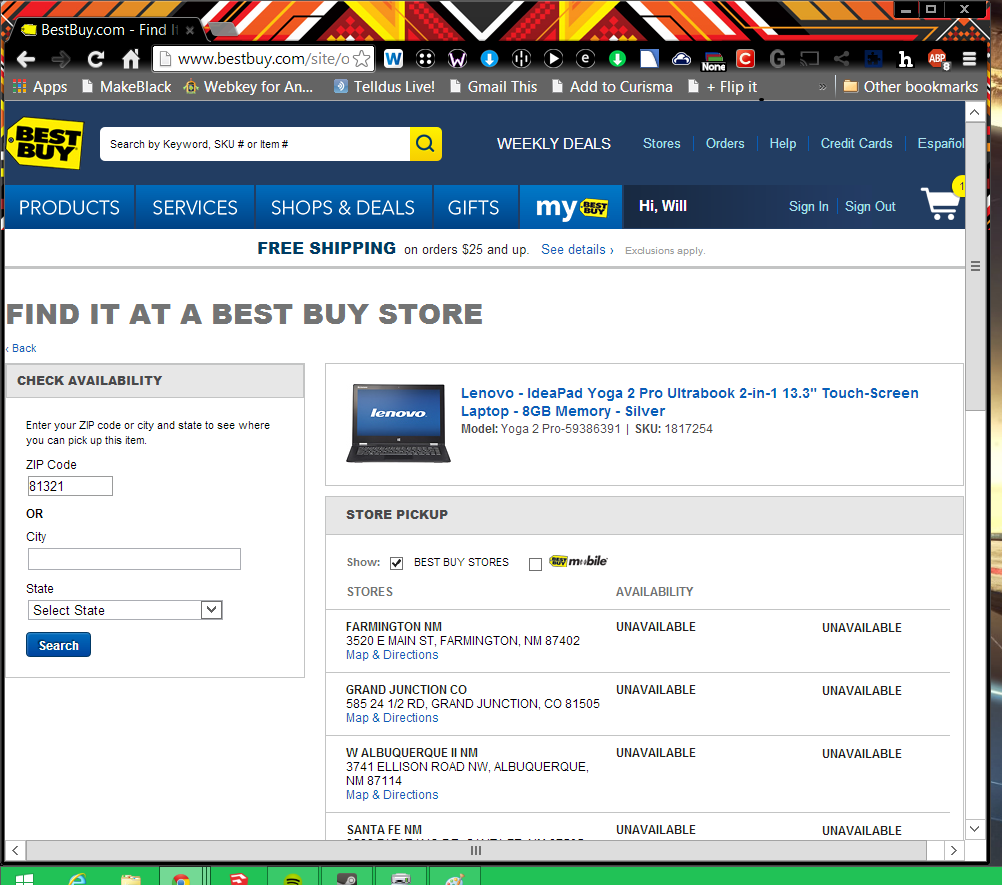This image showcases the Best Buy website interface. 

At the top left corner of the browser window, the familiar Best Buy logo is displayed, featuring a gold-tag icon next to the text "BestBuy.com" with a small gray separator line followed by an 'X' icon. The browser's background is black, incorporating navigation elements such as a left-pointing white arrow, a non-highlighted right-pointing arrow, and a white redo arrow along with a house icon. 

Beneath these navigation tools, the URL bar reads "BestBuy.com" indicating the active website, followed by various top icons typically seen in a browser window.

Under the URL bar, multiple page tabs such as Gmail, Teldes Live, and WebKey are visible. The central part of the web page prominently displays the traditional Best Buy logo next to a search menu.

In the header section, below the logo, a navigation menu starts with "Weekly Deals" and extends rightward, including links to "Stores," "Orders," "Health," "Credit Cards," and "Español." On the left side, another menu features options such as "Products," "Services," "Shop and Deals," "Gifts," "My Best Buy," and personal account links like "Hi Will" with a "Sign Out" option. A shopping cart icon on the right corner shows a small notification with the number '1.'

Underneath these navigational elements, the website promotes free shipping and lists details for finding items at a Best Buy store. A Lenovo computer is prominently displayed as a featured product, including options for store pickup and availability in various regions. Next to this, a "Check Availability" section prompts users to enter their zip code, city, state, and then click the search button to find product availability information.